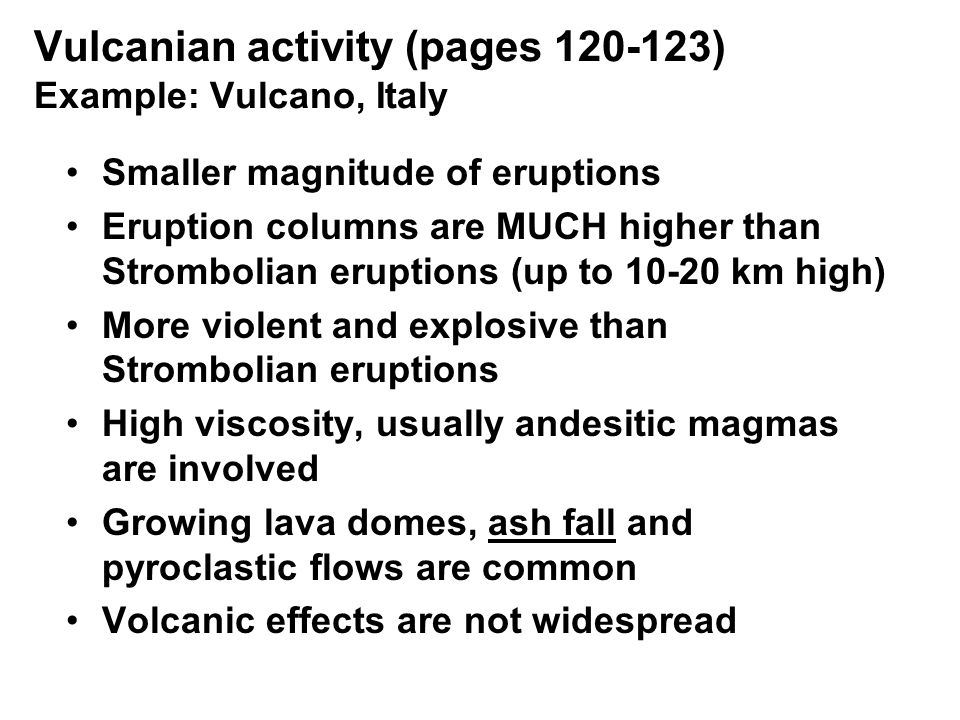The image displays a plain black and white page from a book, titled "Volcanian Activity" at the top, followed by a notation in parentheses, “pages 120-123.” Below the title, it reads, “Example: Vulcano, Italy.” The page features six left-aligned bullet points detailing information about Volcanian eruptions. 

1. Smaller magnitude of eruptions.
2. Eruption columns are MUCH higher than Strombolian eruptions (up to 10 to 20 kilometers high).
3. More violent and explosive than Strombolian eruptions.
4. High viscosity, usually andesitic magmas are involved.
5. Growing lava domes, ashfall (underlined), and pyroclastic flows are common.
6. Volcanic effects are not widespread.

All the text is in black, creating a stark contrast against the white background. The page has a simple, scholarly layout, reminiscent of a textbook.